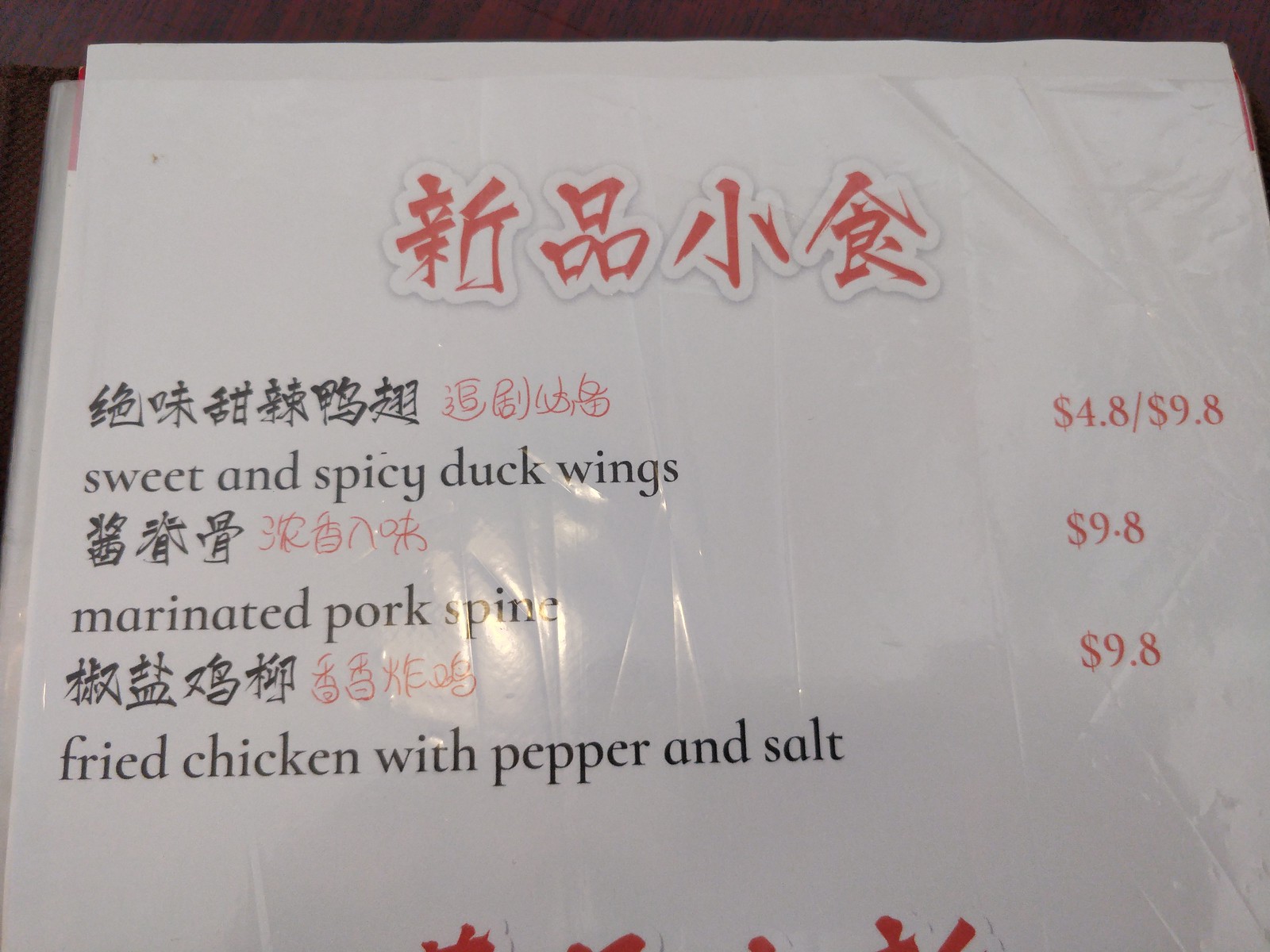This image features a section of a Chinese menu encased in a somewhat wrinkled and scratched clear cover. The menu itself is printed on white paper and showcases three culinary offerings. At the top, red Chinese characters denote the header, while more red characters appear at the bottom, though partially cut off. The menu lists items in Chinese, with English translations provided below each dish name, and the prices highlighted in red along the right-hand margin. The selections include "Sweet and Spicy Duck Wings," available in two sizes priced at $4.80 and $9.80, "Marinated Pork Spine" for $9.80, and "Fried Chicken with Pepper and Salt," also priced at $9.80. The clear cover has visible wrinkles and folds, adding a touch of wear and authenticity to the scene.